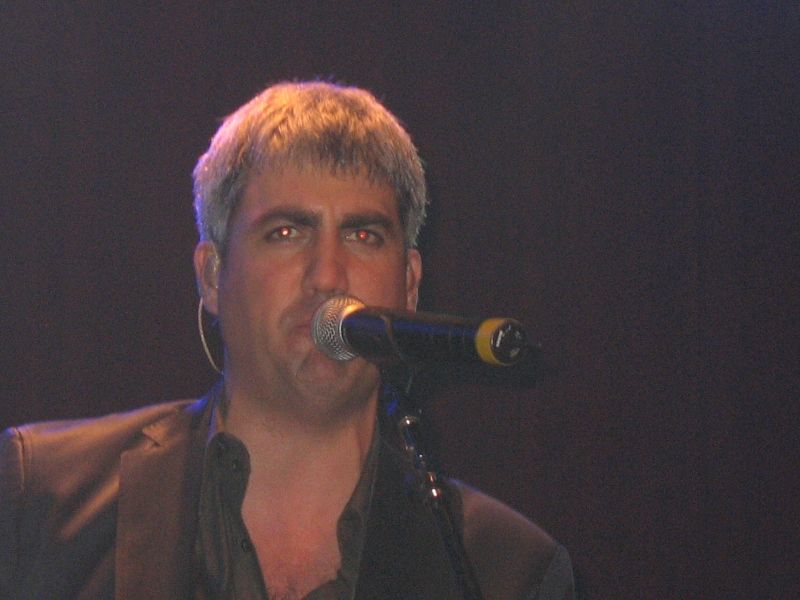This digital photograph captures a middle-aged white male with shaggy, spiky dark gray hair, centered in the image as he sings into a black and silver microphone. He is outfitted in a black button-down collared shirt paired with a black suit jacket. Notably, he has an earpiece in his right ear. The background is a pitch-black expanse, intensifying the spotlight on him, and suggesting a possible nighttime concert or a dark indoor music venue. The overall color scheme includes black, silver, gray, and minor hints of red, gold, and maroon. His eyes appear red due to camera flare.